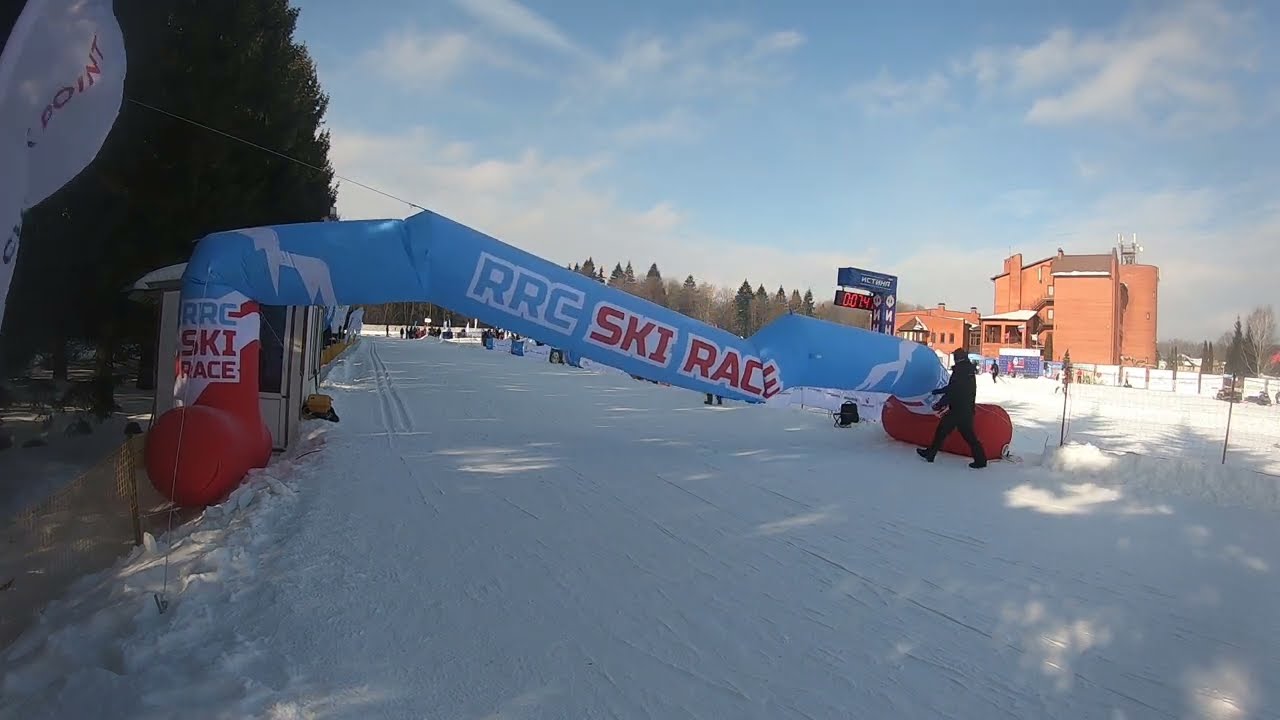In this color photograph taken during the daytime, a snowy racetrack stretches across the scene, framed by a variety of elements that illustrate the cold weather and event setting. The background is dominated by a clear blue sky dotted with scattered clouds and a thick band of clouds along the horizon. In the foreground, the snow-covered ground is packed down to create a raceway. Central to the image is a partially deflated balloon archway with light blue and white colors, emblazoned with "RRC Ski Race." The balloon is anchored by red feet on either side of the track. A man is positioned on the right, struggling to fully inflate the arch, which is connected to orange tanks likely used for inflation.

To the left, a large pine tree stands tall, while more pines are visible farther back along the snowy path. A red brick building with multiple units is visible in the background on the right, providing a stark contrast with its deep color against the snowy and cloudy landscape. An additional detail includes a deflating banner or balloon with the word "point" on it, and a digital timer or scoreboard also appears in the vicinity. The overall palette of the photograph is marked by the blues of the sky and banner, the white snow and clouds, and the greenish-black trees in the background, creating a vivid and detailed portrayal of the race day preparations.